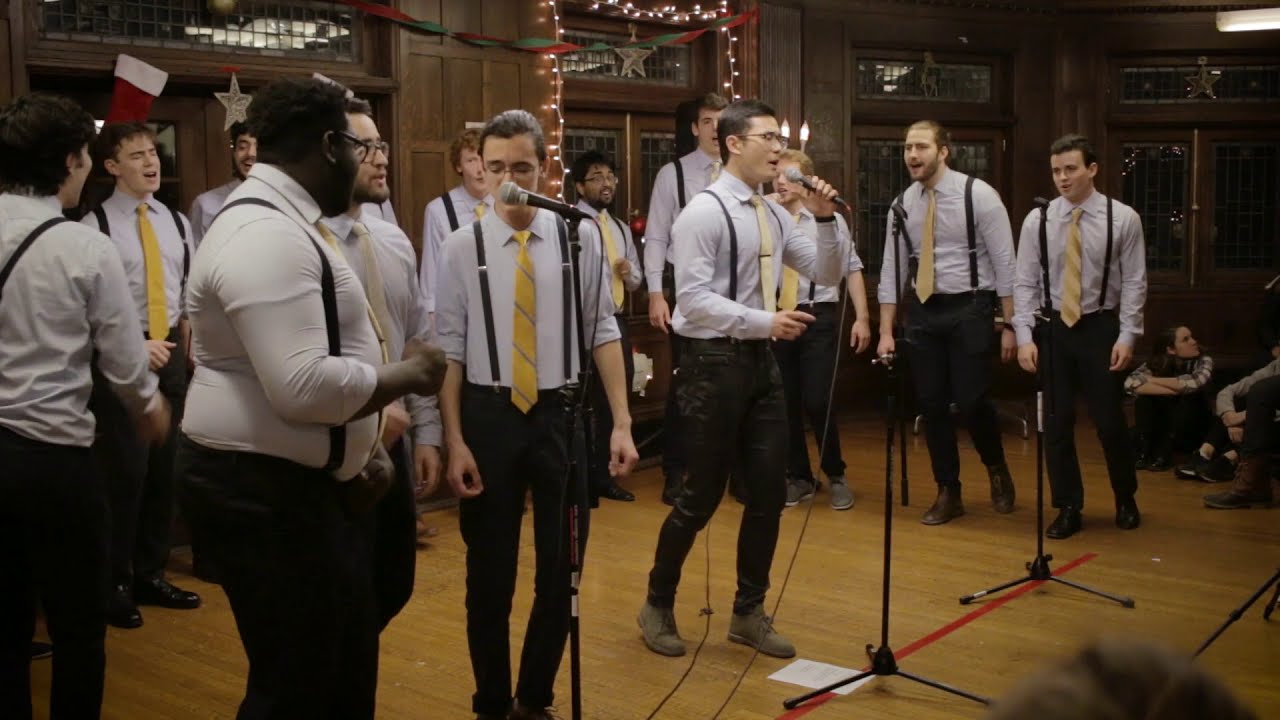The wide rectangular photograph captures a festive a cappella performance inside a warmly decorated room. The floor and walls are constructed of light and dark brown wood respectively, with several visible windows adorned with gold stars above them. Red and green streamers and Christmas lights enhance the holiday atmosphere, and a stocking is hung in the top left corner, adding to the festive decor.

The image features a diverse group of approximately 12 men, standing on a wooden platform that blends seamlessly with the rest of the room. They are dressed uniformly in light blue collared shirts, black pants, suspenders, and yellow ties with thin, widely spaced purple stripes. The men are either standing at three microphones positioned in the front or forming a supportive half-circle around them.

Additional figures can be seen seated on the floor on the right side of the image, dressed in different attire, suggesting an audience or support crew. The focus remains on the singers deeply engrossed in their performance, contributing to the room's vibrant and joyous holiday ambiance.